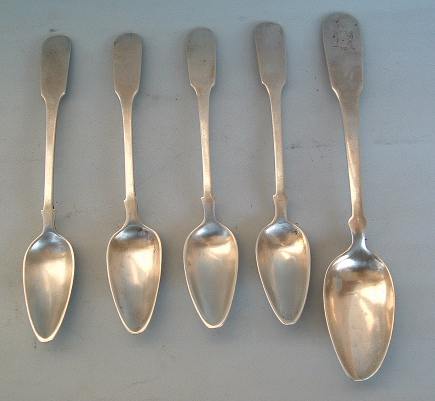The photo depicts a collection of five antique silver spoons arranged across a gray, possibly granite, countertop. The four spoons on the left are of the same size, likely teaspoons, characterized by their small, slightly oval-shaped bowls that taper towards the handle. These teaspoons have narrow handles that widen at the end, and they appear to share a consistent quality and lack distinctive designs at their handle tips. The fifth spoon, situated on the far right, is notably larger – probably a tablespoon – and features a similar shape but on a bigger scale. This larger spoon has a decorative design at the end of its handle and shows some signs of oxidation, including darkness, chipping, and slight holes, indicative of its antique nature. The overall arrangement highlights the contrast between the uniformly sized teaspoons and the more substantial tablespoon.